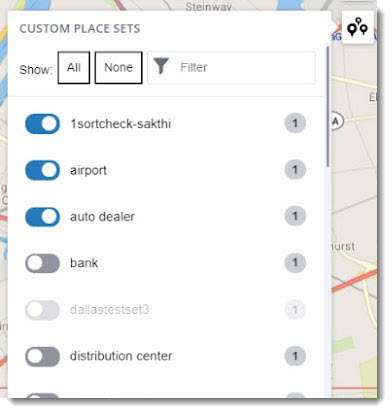### Detailed Caption for the Image

This image is a close-up screenshot of a map interface, possibly from Google Maps or another mapping website. The background showcases a traditional map layout with visible street lines and geographical markers. Overlaying this is a clean, white pop-up window titled "Custom Place Sets." Within this pop-up, there is a range of interactive elements for filtering places on the map.

Notably, at the top of the pop-up, there's a section labeled "Show" accompanied by filter options labeled "All" and "None." Beneath these options is a filter search box for more specific queries. Adjacent to these filters on the left are several toggle switches, each corresponding to an item in a list.

The list of items, aligned horizontally from left to right, consists of toggle switches, descriptive text, and gray circles. Each gray circle contains the number "1" in slightly darker text, with one circle appearing lighter, suggesting it is grayed out. The descriptive text for the items in the list, ordered from top to bottom, reads as follows: "sort check, sat key, airport, auto dealer, bank, Dallas test set three, distribution center," with the final item partially cut off at the bottom of the image.

The entire pop-up window, along with its contents, has a subtle drop shadow effect, indicating it is an overlay element on a web page.